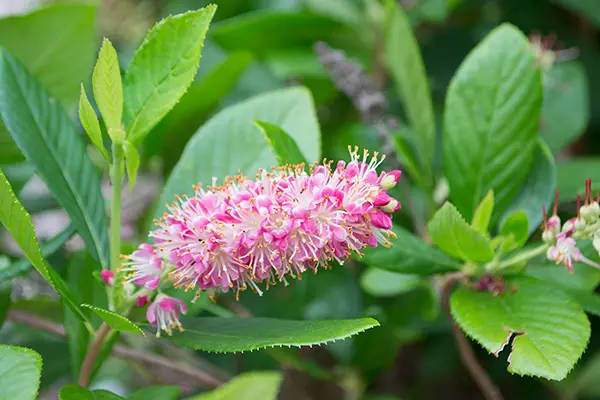The image showcases a vibrant nature shot featuring a prominent flower with multiple elongated blooms, reminiscent of honeysuckles, at the center. The flower exhibits a striking combination of pink and white hues, with pink tips transitioning to white towards the insides. Positioned amidst lush green leaves and foliage, the main flower stands out with several blooms clustered together on a single stem, which also includes shades of purple and brown. Surrounding the central flower are more green plants and blurred leaves in the background, adding depth to the scene. To the right, a secondary stem with nascent pink and white buds—having yet to fully bloom—can be seen. These buds have visible pistils and stamens with small orange tips. Additionally, small, un-sprouted seeds are noticeable at the bottom left. The overall bright daylight setting suggests the photograph was taken looking downward or sideways at the vegetation, capturing the vibrant interaction of colors and details in the natural flora.